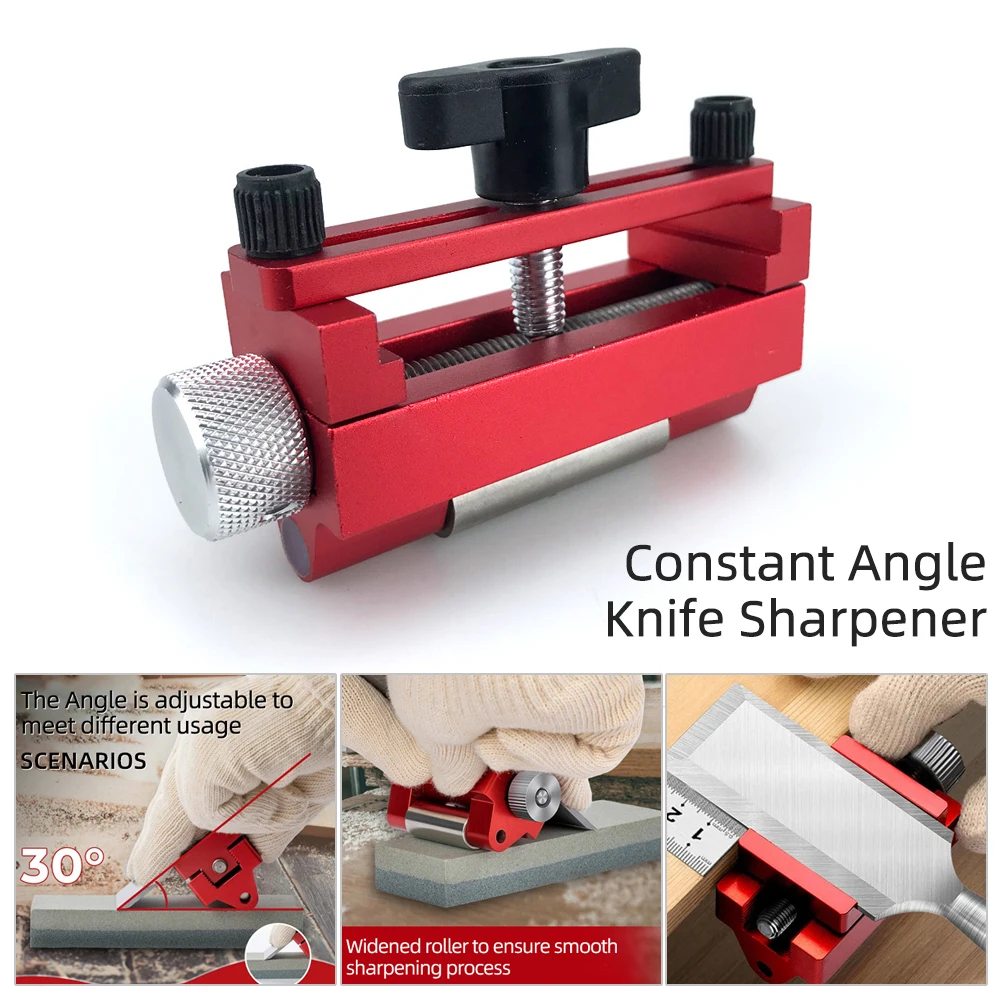Introducing the Constant Angle Knife Sharpener, a robust and compact sharpening device designed for precision and versatility. Made of bright, metallic red metal, it features prominently three black knobs on top and a chrome-adjustable silver knob on the side, ensuring durability and ease of use. The central black knob includes a silver screw for fine adjustments, complemented by intersecting screws on the side knob for stability.

Incorporating a widened roller, the sharpener ensures a smooth sharpening process, accommodating different angles, with a specific example of a 30-degree adjustment. Below the descriptive text, a series of three instructional images provide a step-by-step guide on using the device. The first image highlights the angle adjustment based on usage needs, suitable for various blades. The second image demonstrates how to properly position a knife on the sharpener, showing the whetstone with fine and coarse textures for optimal sharpening. The third image showcases the device's capability to clamp and sharpen a wood chisel, exemplifying its versatility.

This detailed instructional and versatile setup makes the Constant Angle Knife Sharpener an essential tool for achieving razor-sharp blades whether for knives or woodworking chisels.